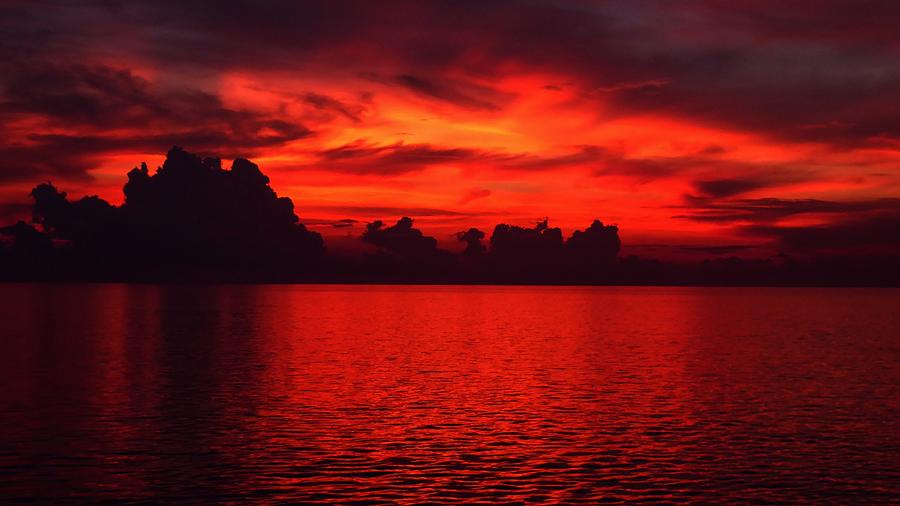In this surreal and likely filtered image, a twilight sky, richly streaked with very dark orange, red, and purplish hues, reflects vividly on a serene body of water. Majestic clouds frame the fiery red and orange sunset, casting dramatic contrasts against the darkening sky. In the distance, craggy hills, possibly resembling an island adorned with tall, tapering trees on the left, fade into smaller formations towards the right. The nearly complete sunset casts a mesmerizing, reddish glow on the rippling water, adding to the ethereal atmosphere, where dark forms of trees or possibly clouds are mirrored on the lake’s surface, enhancing the otherworldly effect.